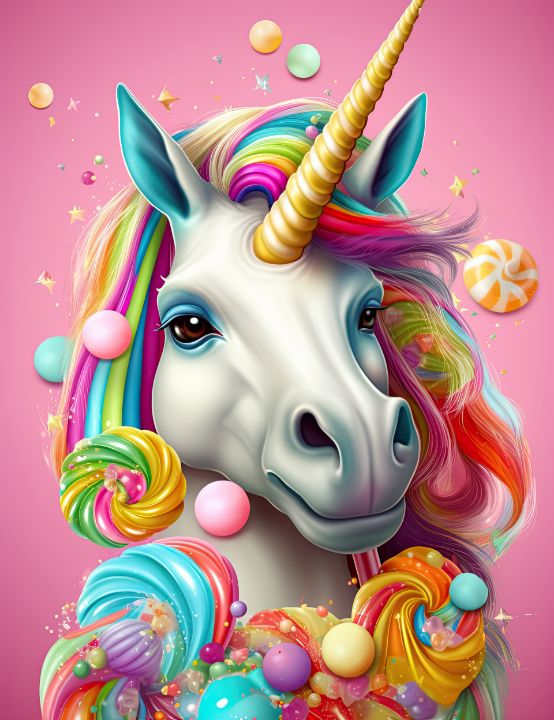The image is a horizontally aligned, digitally generated or hand-drawn illustration depicting a whimsical unicorn with a distinct, intricate design. The unicorn, occupying the left side of the rectangular frame, is shown from the chest up, standing on its hind legs. It has a pristine white face and body, accented with a long, spiraled horn that points up and to the right, featuring alternating yellow and white stripes. 

The unicorn’s mane is a lavish cascade of multicolored hair, swirling around its head and chest, with shades of yellow, green, purple, pink, blue, and orange. Its long ears are white on the outside with blue inner linings. The eyes are bordered in blue, adding emphasis to its expressive black eyes, and blue also accents around the nostrils. The chest is adorned with multicolored curls and swirls, featuring prominent hues of yellow, red, blue, and purple. 

Floating around the unicorn are various small, round balls in colors such as yellow, gold, purple, and teal, some of which might be mistaken for candies due to their shape and color. Specifically, beneath its snout is a purple ball, with a yellow ball slightly above and to the right. In the upper right area of the image, there is an orange and white nautilus-like object, adding to the playful scenery. Behind the unicorn, its luxuriant hair transitions into a liquid-like purple pool, with gentle ripples forming waves. Further in the background are additional vibrant details, possibly a landscape or more elements of the mane, with colors like green, red, pink, blue, and purple encircling the area.

The background of the image is a gradient of pink with a slight purple tinge, becoming lighter towards the center, suggesting a light source from the left center. Scattered throughout the scene are stars and multicolored candies, enhancing the picture's magical and child-friendly aesthetic.